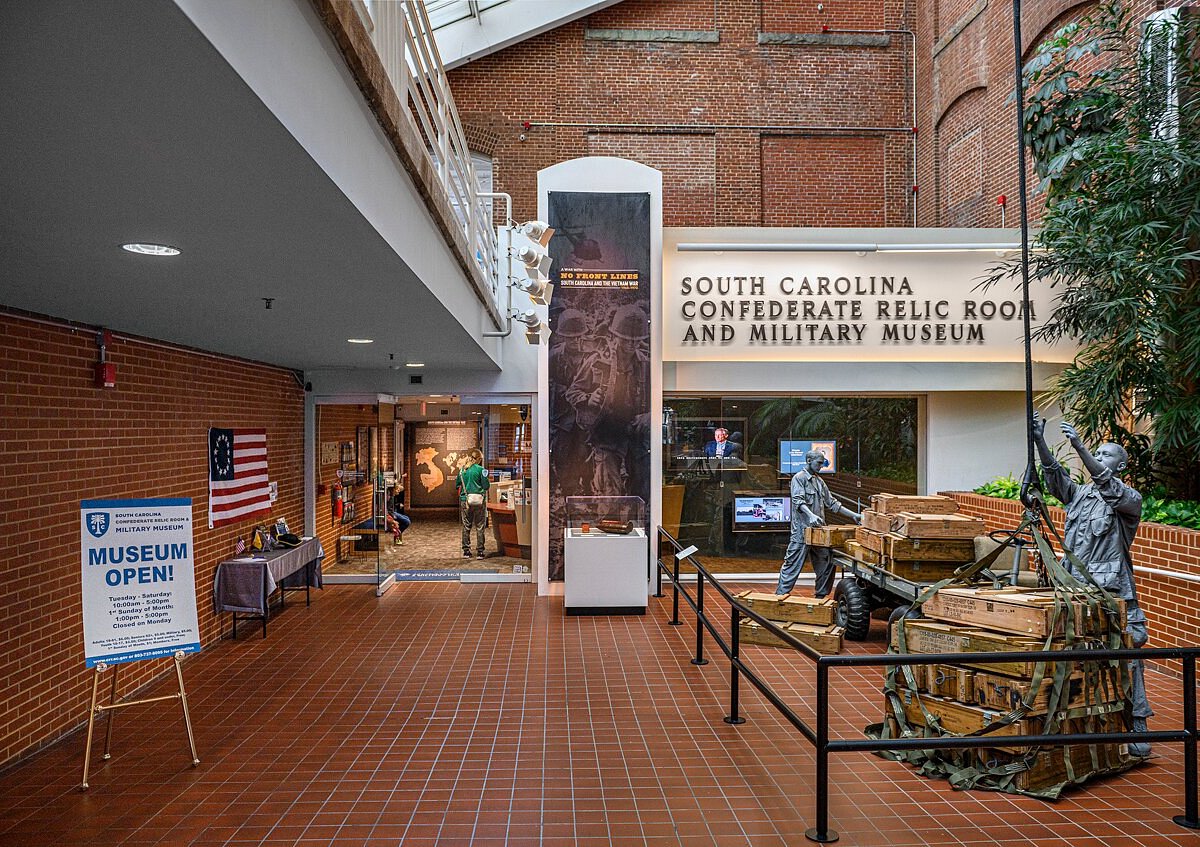The image depicts the entrance hall of the South Carolina Confederate Relic Room and Military Museum. Centrally located in the shot is a glass door leading into what appears to be a reception area. Prominently displayed on the right is a sign and a poster board, both announcing the museum's name and hours of operation: open Tuesday through Saturday from 10 a.m. to 5 p.m., and on the first Sunday of the month from 1 p.m. to 5 p.m., while being closed on Mondays.

The room features several notable elements, including brick walls and skylights that add to the inviting atmosphere. An old American flag with 13 stars in a circle hangs prominently, complemented by a modern American flag adorning a brick wall. 

A fenced-in area catches the eye, showcasing statues of soldiers in action, one of whom is loading crates onto what could be an army truck, possibly even a helicopter based on the context. Behind this area, glass windows reveal TV monitors and screens likely displaying documentaries and interactive exhibits related to the Civil War and the Vietnam War, as indicated by a banner reading "No Front Lines, South Carolina and the Vietnam War." 

Adding to the historical ambiance, there is a monument with figurines dedicated to troops, as well as other relics that provide a deep dive into military history. The overall scene is one of rich historical narrative, blending artifacts, engaging displays, and a respectful nod to the past.